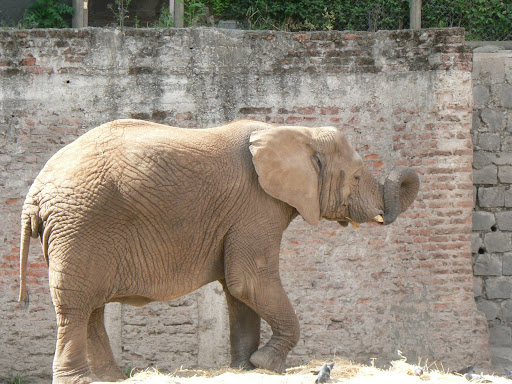In this detailed photograph, a young, dark tan elephant stands prominently in the center of an outdoor enclosure, which appears to be part of a zoo. The elephant, facing to the right, has its right front leg slightly raised. Its trunk is curled around one of its emerging, small white tusks, giving it a dynamic posture. The ground of the enclosure is a mix of grass, dirt, and various types of brush. Dominating the background is a tall brick wall, approximately 10 feet high, transitioning from red at the bottom to darker hues towards the top, suggesting aging or weathering. To the right, this brick wall connects to a taller stone wall composed of larger, tan-colored stones. Beyond these walls, tree trunks are visible, indicating a natural setting surrounding the enclosure. The photograph is richly colored with shades of green, brown, gray, tan, red, and maroon, and captures the scene in broad daylight, heightening the vividness of the outdoor environment.